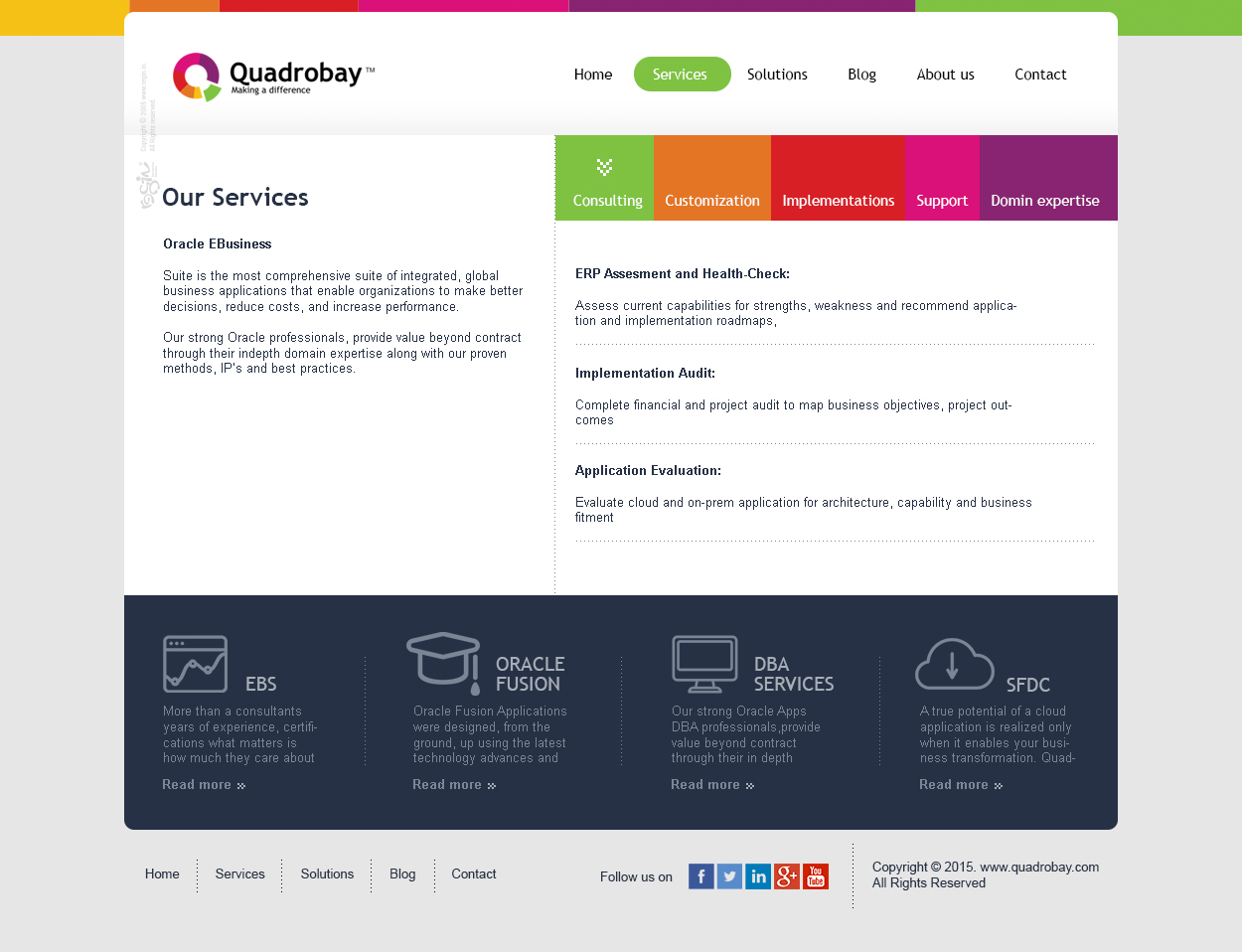Here is a more detailed and cleaned-up caption based on the provided description:

---

The image features a vibrant and structured layout with a rainbow-like color scheme. Starting from the left and moving to the right at the very top, the colors are: yellow, orange, red, pink, purple, and finally green. Below this colorful arrangement is a prominent circle segmented into four quadrants, each filled with different colors: pink, purple, green, and yellow. 

To the right of the circle is the bold text "QUADROBAY." Following this, there is a horizontal menu displaying various options: "Home," "Services" (highlighted within a green circle), "Solutions," "Blog," "About Us," and "Contact."

Moving downward, there is an organized color-coded list, each item contained within a colored box:
- A green box labeled "Consulting"
- An orange box labeled "Customization"
- A red box labeled "Implementation"
- A pink box labeled "Support"
- A purple box labeled "Domain Expertise"

On the left side, written in black text, are the headers "Our Services" and "Oracle E-Business." Toward the bottom, a long dark gray box contains the abbreviation "EBS," and next to it is an image of a square intersected by a line. Below this, there is an image of a graduation cap beside the text "Oracle Fusion." Further down is an image of a laptop, next to the label "DBA Services." Finally, there is an image of a cloud with a downward-pointing arrow inside it, next to the uppercase text "SFDC."

The entire layout is visually structured to provide an effective overview of various services and options.

---